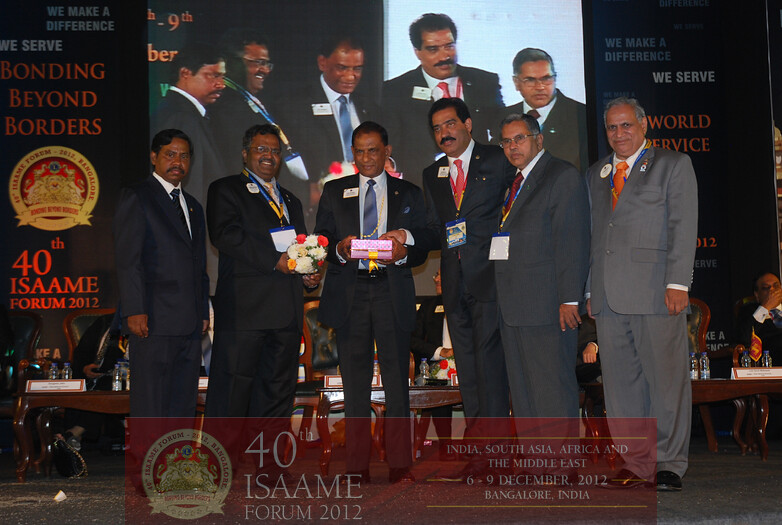The image captures a significant moment at the "Bonding Beyond Borders, 40th Issam Forum 2012" event held from December 6 to 9, 2012, in Bangalore, India. Six Indian men, all dressed in formal suits and ties—five in black suits and one in a dark gray suit—stand on a stage. These men are part of an award ceremony, each holding different items: the man in the middle proudly holds up a trophy, and the man to his left cradles a bouquet of flowers. Most of them are wearing identification lanyards or name cards. Three of the men sport mustaches, while the other three are clean-shaven. Behind them, a large screen projects their live image to the audience, giving the impression that the proceedings are being recorded or teleprompted. The screen displays text on the left, reading "Bonding Beyond Borders, 40th Issam Forum 2012," and on the right, the phrases "We Make a Difference, We Serve." Below the stage, a banner reiterates the event details: "40th Issam Forum 2012," and lists the regions of focus—India, South Asia, Africa, and the Middle East—underscored by the event’s red backdrop with gray or white text. The setting suggests a prestigious platform celebrating accomplishments within these global communities.